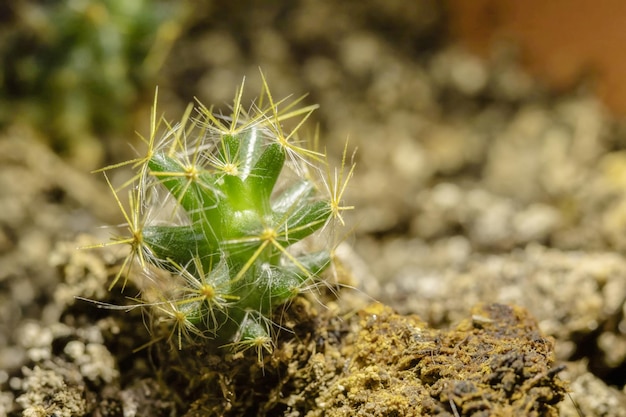This photograph captures a bright, vibrant green cactus in a close-up shot that dominates the composition. The tiny cactus, adorned with dull yellowish spines at each tip, stands out vividly against a backdrop of blurred grays and dull greens. The spines, sharp yet delicate in appearance, extend from the cactus in a spiral pattern, emphasizing its small size as they seem disproportionately large. It is nestled on what appears to be a mixture of dark grayish or brownish gravel, potentially covered with moss or dirt, adding texture to its base. The overall setting is ambiguous—whether it’s in a garden or out in nature remains unclear—but the focus on the cactus creates an intimate, detailed view of this tiny, resilient plant. In the background, hints of other rocks or possibly another distant cactus add depth to the scene.